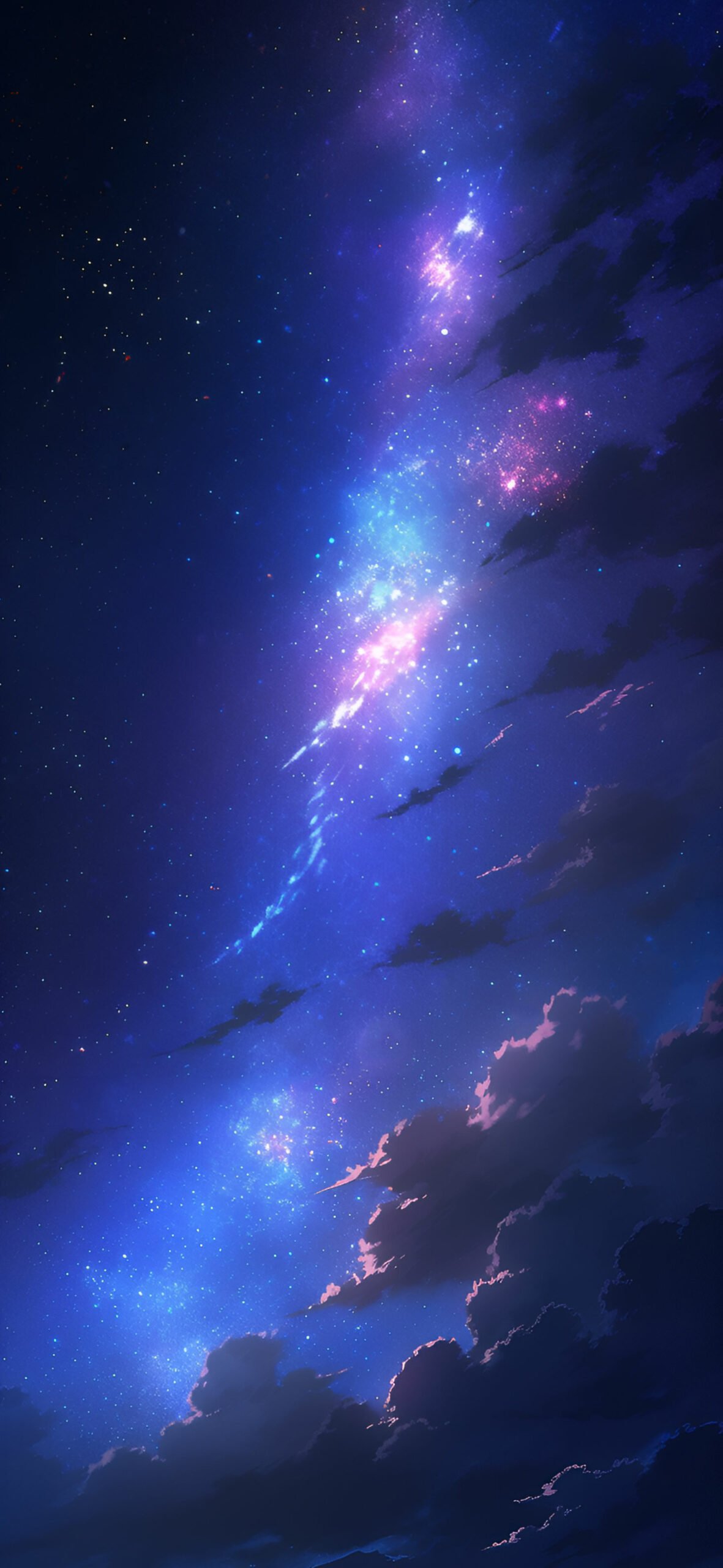This detailed portrait-oriented color illustration depicts a dramatic nighttime sky scene created by an artist. The image showcases an interplay of light and darkness, manifesting in jagged clouds and vibrant hues. The left-hand side of the sky starts with an almost black region at the top left corner, scattered with tiny stars of various colors, including blue, yellowish-white, and red. This dark sky transitions towards a medium and eventually a brighter blue hue as it moves downward.

Dominating the center of the image is an irregular column of nebula-like light that cascades from the top to the bottom. This striking central area features a mix of vivid pinks, purples, and blues. The bright central light source has pink highlights, with a concentration of pink stars in the heart of the image, contrasting against light blue and white highlights around other stars.

Intruding from the right side are dark, jagged clouds that grow larger towards the bottom, eventually stretching across the width of the image. These clouds, nearly black in color at the top, reflect the central light source with lighter pink edges near the bottom. Additional darker pink-edged clouds appear at the very base.

Overall, this tall and narrow painting, more than twice as tall as it is wide, presents a fantastical and richly colored skyscape teeming with artistic imagination, seamlessly blending cosmic elements and dark clouds with vibrant highlights and scattered stars.